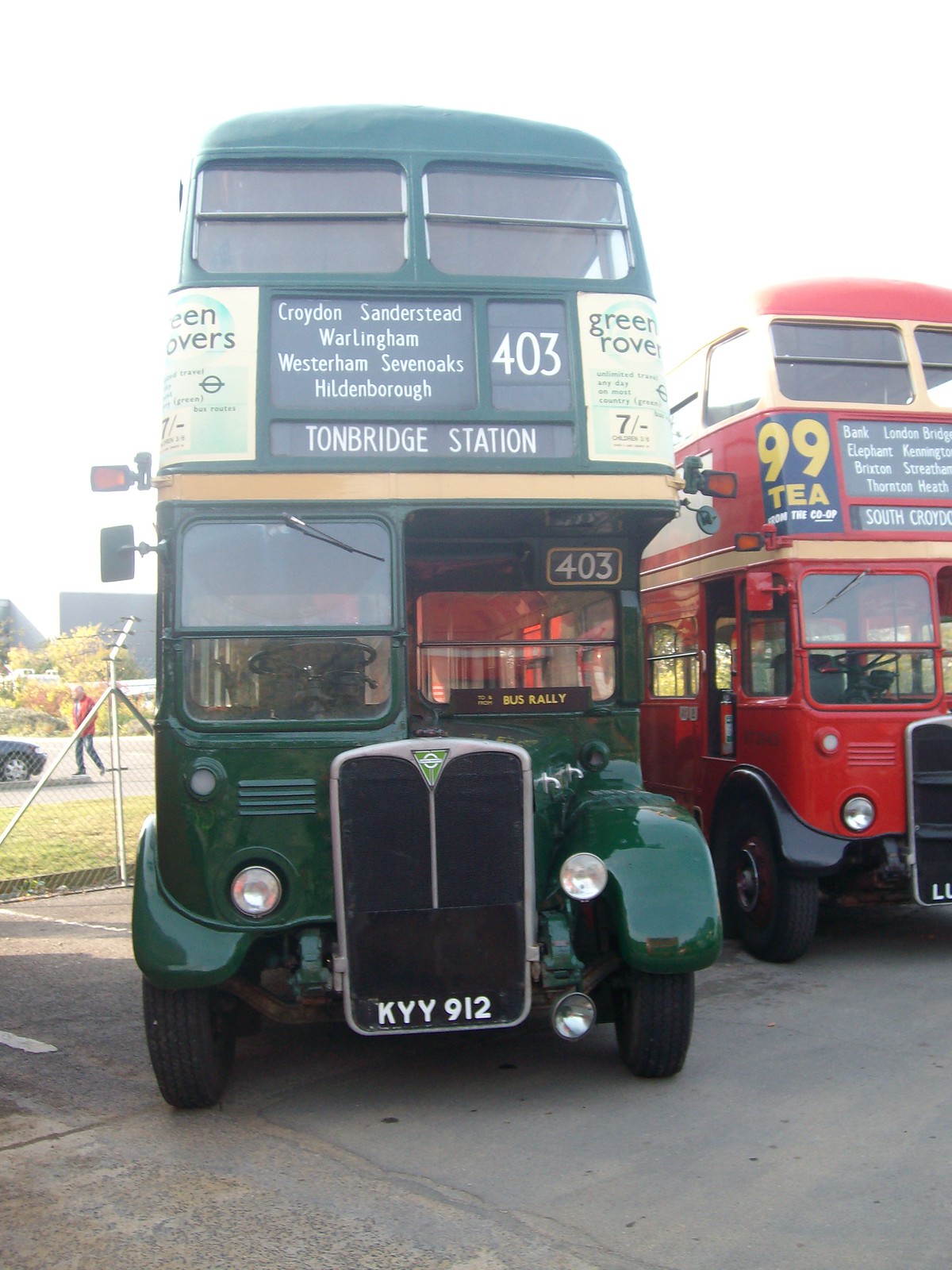In the image, there are two very old, double-decker school buses parked in what looks like a parking lot area. The bus on the left is green and the bus on the right is red. The green bus features several textual details: on the lower front, the license plate reads "KYY 912," while the upper right front windshield displays the number "403." Higher up, on the second story of the green bus, white text lists locations: "Croydon, Sanderstead, Warlingham, Westerham, Sevenoaks, Hildenborough, Tonbridge Station." Below these details, there is another "403" plate and to the right side, an additional sign reads "Green Rover." The red bus also has words at the top indicating stops, and on its upper corner, there's a sign that says "99T, T-E-A." Behind the green bus is a chain-link fence, and through it, you can see the front end of a car and a person.